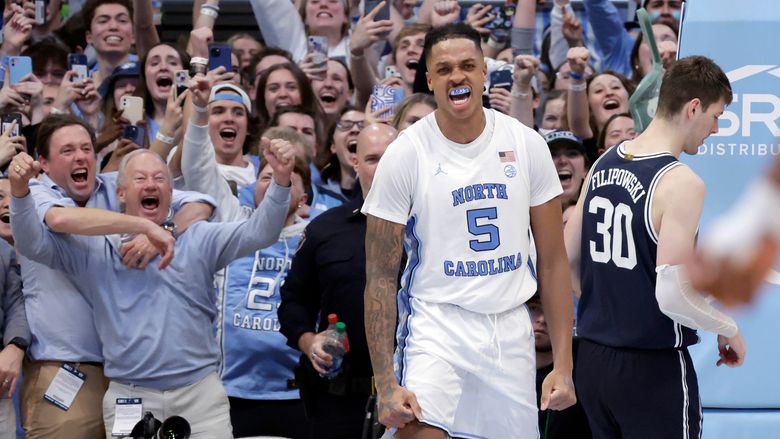The image captures a vibrant moment at a home college basketball game, featuring a North Carolina player centered prominently. The player, sporting a white North Carolina jersey with baby blue accents and the number five, stands out with a Jordan logo and an American flag patch over his heart. He has tattoos on one arm and wears a mouth guard, a short-sleeved shirt underneath his jersey, and matching shorts. To his right stands an opposing player, likely named Filipowski, wearing a dark blue or black jersey with white lettering and the number 30.

Surrounding the players is an energetic crowd, predominantly dressed in North Carolina gear, indicating a home game atmosphere. Fans fervently cheer and capture the moment on their phones. Notably, in the bottom left corner, two enthusiastic spectators can be seen; one man wraps his arms around another, who has his arms raised in excitement. The photograph, taken from court level, effectively conveys the intensity and excitement of a college basketball game.